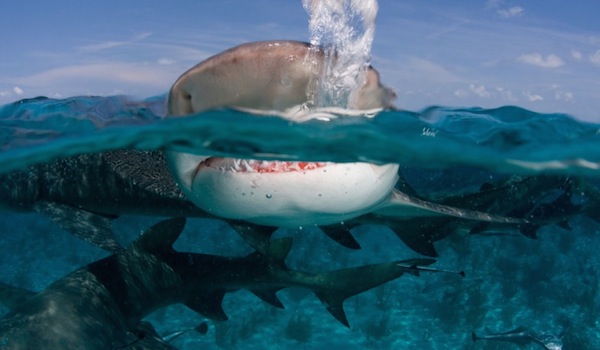The image captures a striking underwater and above-water scene featuring a majestic marine creature. Dominating the center, a large shark, colored gray on top and white on the bottom, emerges partially from the water, releasing bubbles from its open mouth. Water sprays around its body as it breaks the surface. The shark’s long fin on its right side is clearly visible. Below it, the dark, shadowy water reveals at least three other fish, including a large one with many fins. The atmosphere is intense with the sky above showing a tranquil blue with sparse clouds, contrasting sharply with the dark abyss below. A faint pinkish section is visible near the shark’s mouth, hinting at its recent activity.